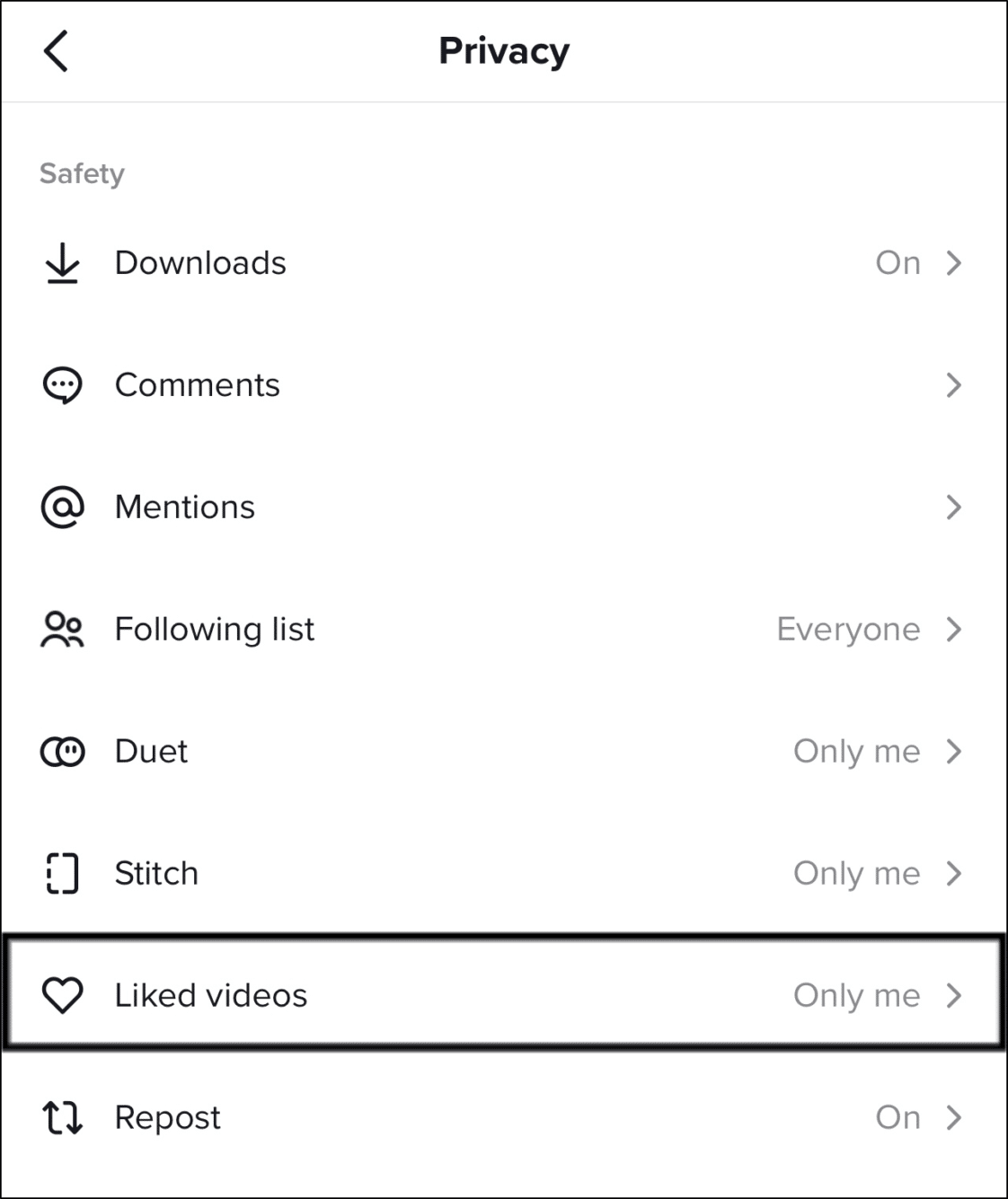The image is a screenshot featuring a user interface with a white background. On the left, there is a left-facing arrow indicating a back function. The screen lists several settings related to privacy and safety, each followed by right-facing arrows. The options on the screenshot are as follows:

- **Downloads** – next to this label is the word "On" followed by a right-facing arrow.
- **Comments** – next to this label is a right-facing arrow.
- **Mentions** – followed by a right-facing arrow.
- **Following list** – labeled with "Everyone" followed by a right-facing arrow.
- **Duet** – labeled with "Only me" followed by a right-facing arrow.
- **Stitch** – labeled with "Only me" followed by a right-facing arrow.
- **Liked videos** – labeled with "Only me" and features a heart icon next to it, followed by a right-facing arrow. This line is highlighted by a black rectangle around it.
- **Repost** – labeled with "On" followed by a right-facing arrow.

This detailed list allows users to manage their privacy and interaction settings comprehensively within the interface.